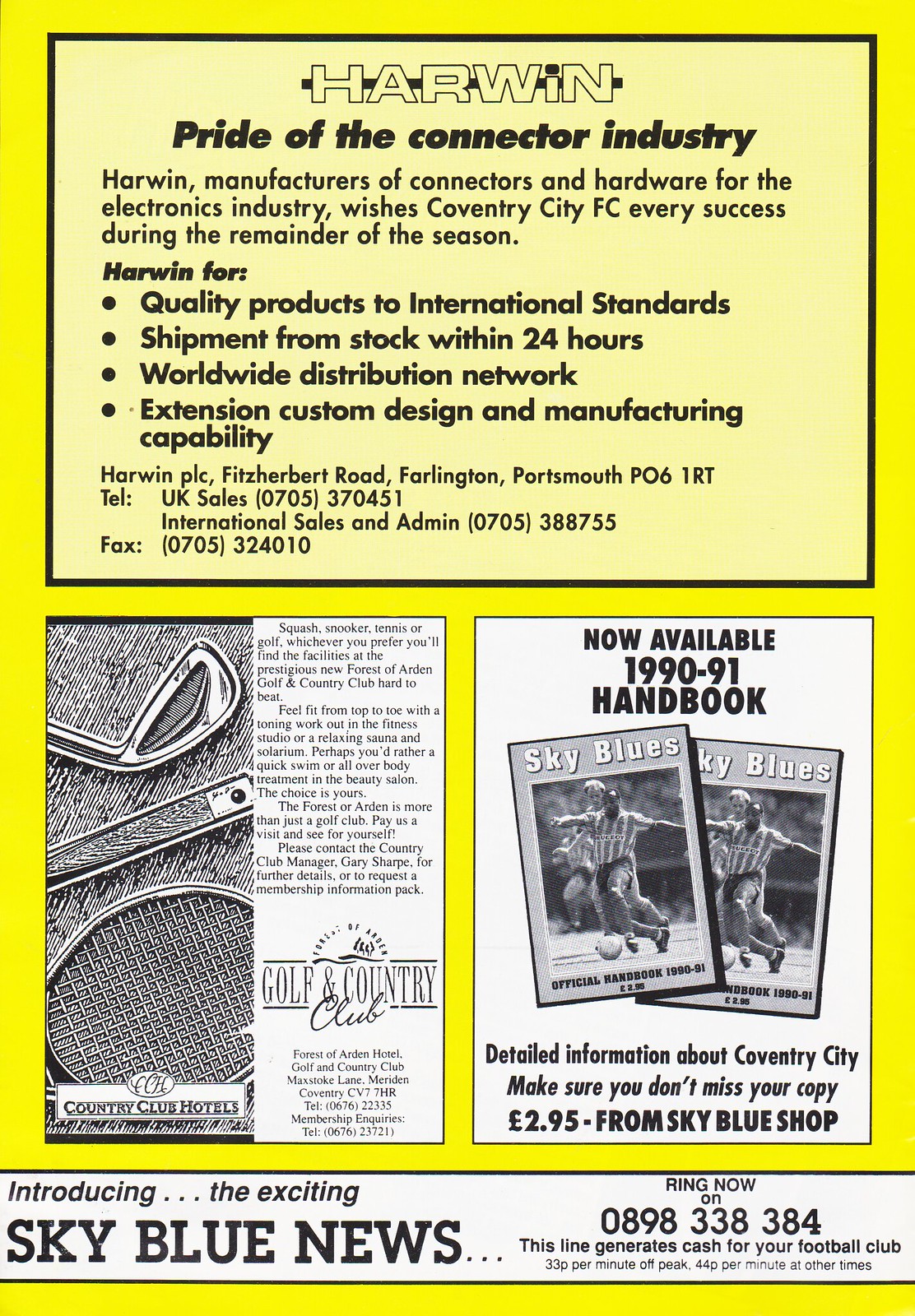This image showcases a page from a soccer program, predominantly featuring an ad for Harwin, the "pride of the connector industry." The Harwin ad spans the top half of the page, displaying a vibrant yellow background with a black border. The ad text, in bubble letters and bold italics, highlights Harwin's role as manufacturers of connectors and hardware for the electronics industry, wishing Coventry City FC success, and detailing their quality products, international standards, 24-hour stock shipment, worldwide distribution network, and custom manufacturing capabilities. Harwin PLC's address and contact information are also included: Fitzherbert Road, Farlington, Portsmouth P061RT, with phone numbers for UK sales and international sales.

In the lower left corner, there’s a black and white ad for the Coventry Golf and Country Club, featuring illustrations of a golf club and a tennis racket. Adjacent to this, in the lower right corner, is an ad for the 1991 Coventry City football handbook, priced at £2.95, available from the Sky Blues shop, with a promotional line for Sky Blues News, a paid hotline for club updates, costing 33p per minute off-peak and 44p per minute at other times, emphasizing that the line generates revenue for the football club.